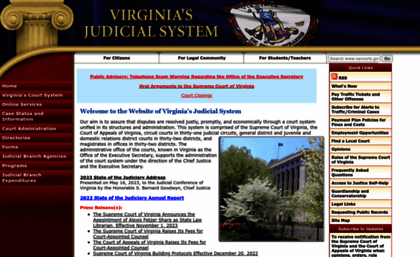This image depicts the homepage of Virginia's judicial system website. At the top, there is a header indicating that it is indeed the official site. Directly beneath the header are various navigation tools. A vertical red sidebar on the left contains ten navigation buttons, but due to the low resolution of the image, the white text on these buttons is illegible. The main body of the page features large text that reads "Welcome to the website of Virginia's Judicial System" with a reference to the "2022 Judicial Annual Report." However, many smaller fonts are also unreadable because of the poor resolution.

The middle part of the page includes a photograph of a building surrounded by white blooming trees, adding a touch of natural beauty. On the right side of the page, there's another list of navigational options, less visible due to the pixelated quality. The website's visual palette includes a variety of colors: red, white, blue, yellow, cream, black, pink, and orange, which are used in text, backgrounds, and graphics throughout the site.